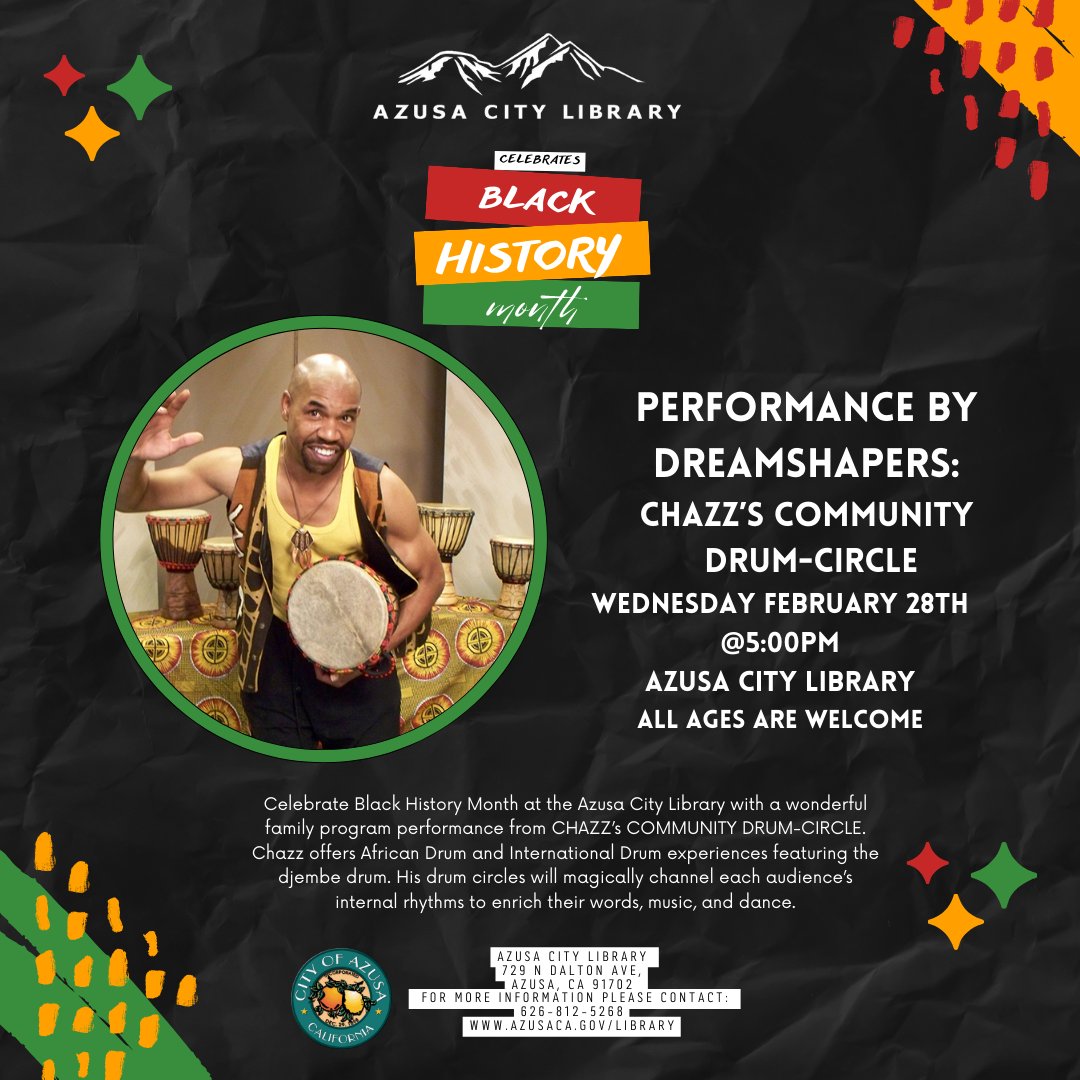The advertisement showcases a drum exhibition event presented by the Azuka City Library, set against a dynamic background designed to catch the eye. The primary backdrop is a textured black and gray, resembling rock or granite, creating a striking canvas for the event details. In the upper section, a black and white illustration of mountains frames the text "Azuka City Library," followed by the celebration announcement for Black History Month, presented in alternating white and bold colors (red, yellow, blue, and green) for emphasis.

Decorative elements further enhance the visual appeal: three colorful stars (red, blue, and yellow) in both the upper left and bottom right corners, and vibrant stripes adorned with multiple dots (yellow stripe with red dots in the upper right, and blue stripe with yellow dots in the bottom left).

A central focal point features a photograph of a smiling man captured mid-performance, holding a bongo drum in his left hand, poised to strike it with his right. The man, dressed in a white sleeveless shirt, black pants, and a vest or backpack, stands in front of a table displaying additional drums with a circular-patterned tablecloth.

Text details the event specifics: "Performance by Dream Shapers: Chaz's Community Drum Circle," scheduled for Wednesday, February 28th at 5 p.m. at the Azuka City Library. The right-hand text block invites “All Ages” to join and celebrates Black History Month with Chaz's unique African and international drum experiences using the Djembe drum, promising an enriching performance.

The bottom of the advertisement provides the library's address, 729 North Dalton Ave, Azuka, CA 91702, and contact information (626-812-5268) along with the library's website (www.azukaca.gov/library), ensuring all interested participants can easily find additional details.